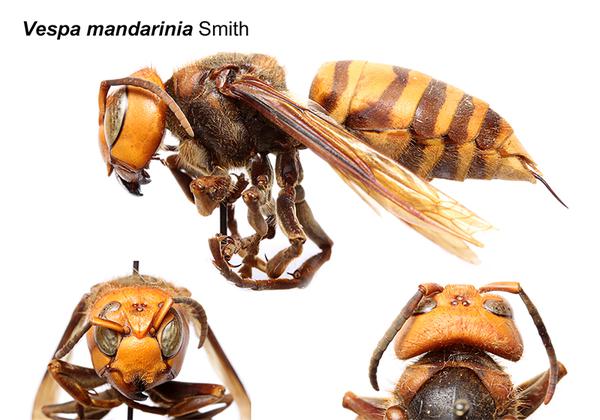This digital drawing features multiple views of a Vespa mandarinia Smith, commonly known as the Asian Giant Hornet. At the top of the image, a side-view illustration of the hornet captures its distinctive orange face, dark and orange-striped abdomen with an exposed stinger, brown legs, and semi-transparent wings. Below this, on the left, a zoomed-in frontal view highlights the hornet's angry expression, silver eyes, brown antennae, and orange face. To the right of the front view, another illustration shows the hornet from an underside angle, displaying its black and golden underbelly. The name "Vespa mandarinia Smith" appears in the upper-left corner in bold italics, with "Smith" in regular font, indicating the scientific classification of the insect.